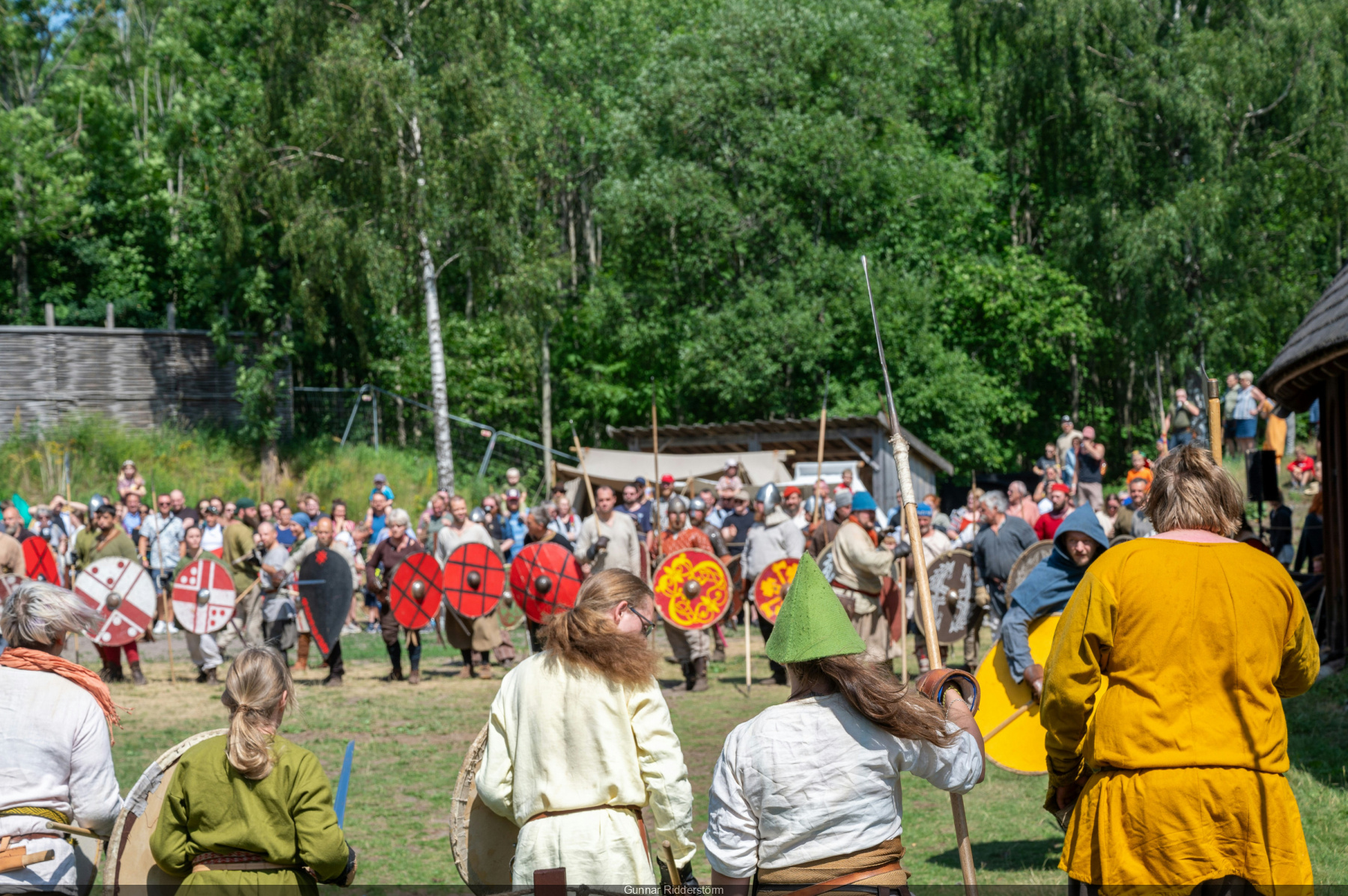In this outdoor photo, a group of people is gathered in a large, grassy field with brown, green, and beige hues. The scene is set against a backdrop of tall, lush, green deciduous trees. To the right, there is a metal shed with a sloped roof, and a series of fences climb up a hill to the left. A makeshift tent is suspended from a rope tied between two trees.

In the foreground, five individuals with their backs turned are equipped in medieval-style attire. On the far right, one person stands out in a bright yellow smock. Next to them is a shorter individual wearing a green cone hat and holding a large spear. At the center, a lady in a white smock holds a brown shield. Another person in a green shirt wields a large circular shield and a blue stick, while a partially cut-off individual stands beside them. 

Facing this group is a larger crowd, including rows of people equipped with circular wooden shields. Among them, various colors and designs can be seen, including red, white, and yellow shields. Some of these participants wear steel helmets with nose guards and carry longswords, suggesting a medieval reenactment. Onlookers in casual clothing stand on a bank observing the event, adding to the scene's dynamic feel. This gathering appears to be a well-attended event with at least a hundred people participating in or watching the activities.